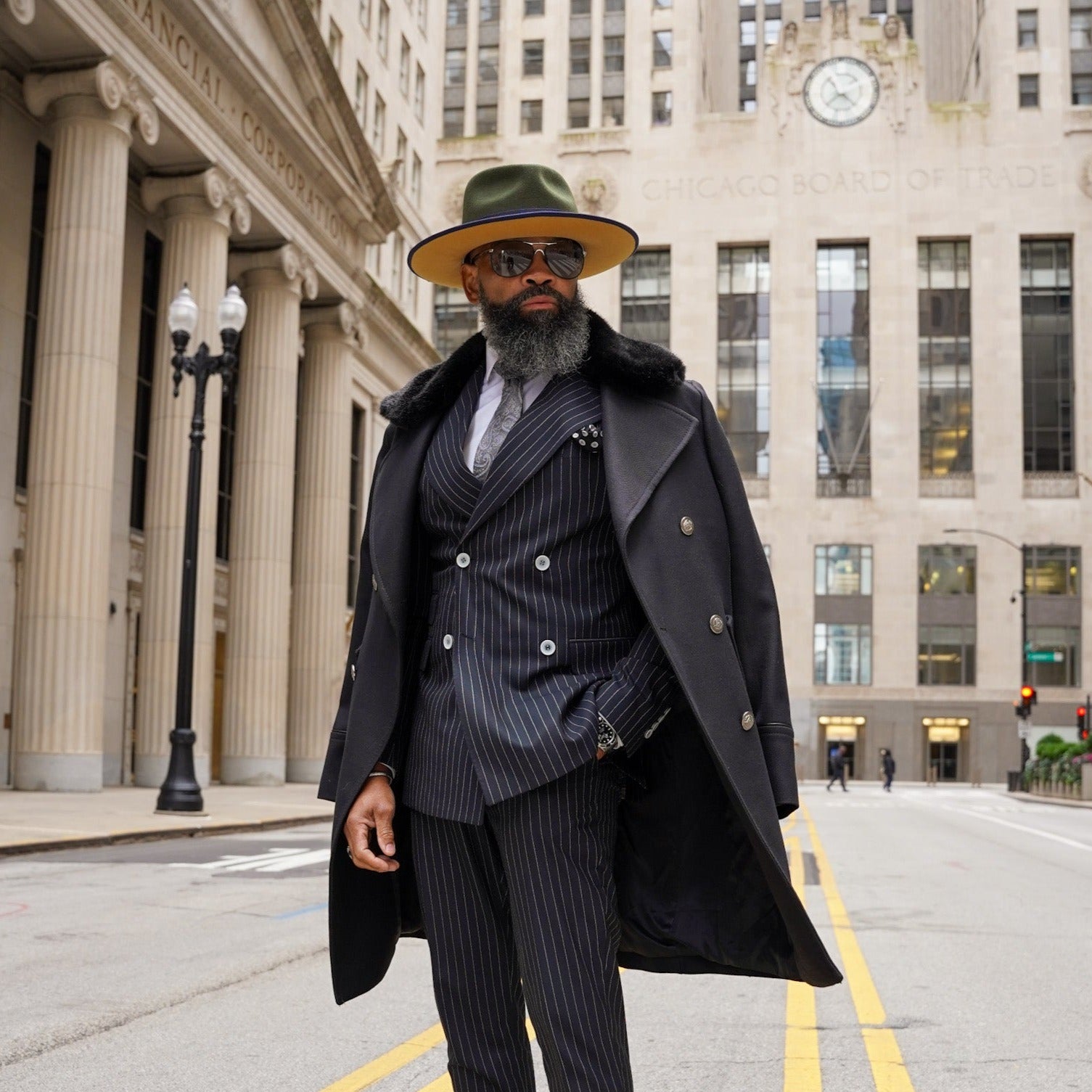This is a detailed photograph of an African-American man who appears to be modeling stylish clothing in an urban setting. He has a salt-and-pepper beard and is wearing a green wide-brimmed hat with a yellow underside. The man is dressed in a black suit featuring a pinstriped pattern in black and gray, with shiny black dress shoes. Draped over his shoulders is a dark overcoat with a distinctive black fur trim around the collar. He completes his look with sunglasses, and his pose is confident, with his left hand casually placed in his pants pocket while his right hand hangs at his side. 

The background reveals that he is standing outdoors in front of the Chicago Board of Trade. This recognizable building showcases tall windows and a prominent clock at the top of its façade. The inscription "Chicago Board of Trade" is clearly visible below the clock. To the man's right, another building with beige pillars bears the inscription "Financial Corporation" above the entrance. The setting appears to be a daytime picture, with a gray asphalt road marked with yellow traffic indicators adding to the urban ambiance.